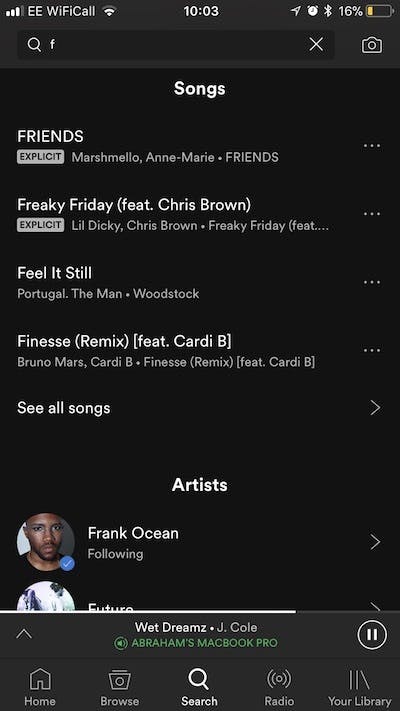The image showcases a page on a user's smartphone. The background is entirely black, with all the text displayed in either white or light gray. 

At the top of the screen, status icons show signal bars, the "EE Wi-Fi call" indicator, the time (10:03), an active alarm, and the battery level at 16%. Below this status bar, there is a search bar that contains a lowercase 'f', an 'x' to close the search bar, and a camera icon on the far right.

In the main content area, white text prominently displays the word "SONGS." The first song listed is "FRIENDS," written in all capital letters, followed by a gray "explicit" label. The artists for this song are Marshmello and Anne-Marie. 

The second song is "Freaky Friday," featuring Chris Brown. This listing also includes an "explicit" label and the artists Lil Dicky and Chris Brown.

The third song is "Feel It Still" by Portugal. The Man, from the album "Woodstock."

The fourth song is "Finesse (Remix) [featuring Cardi B]," with smaller gray text underlining that it’s by Bruno Mars and Cardi B.

Below these song listings, white text reads "See all songs."

Further down, in bold white text, the section labeled "ARTISTS" appears. The first artist listed is Frank Ocean, with an indication that the user is following him.